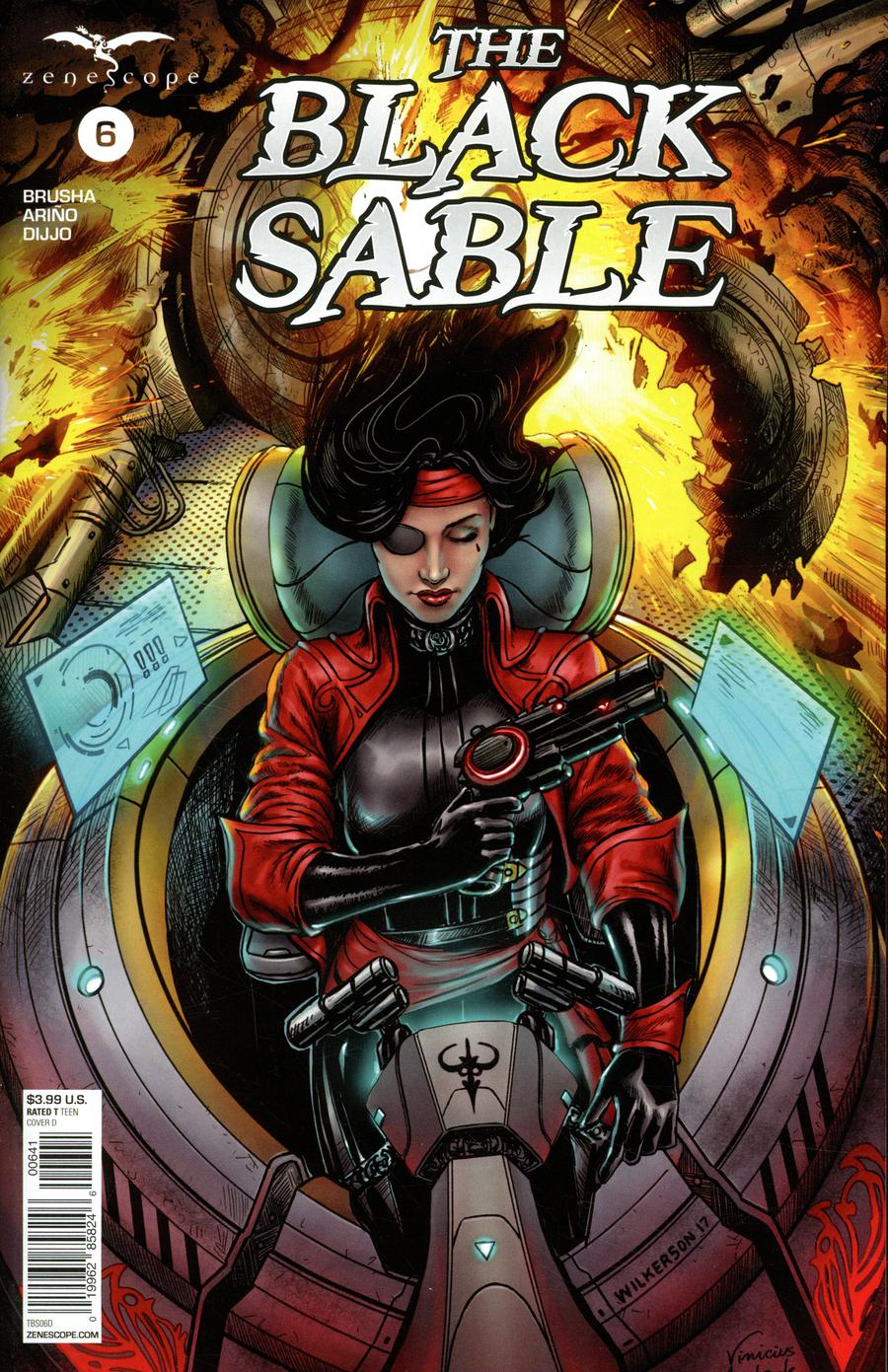The comic book cover art for "The Black Sable" showcases a dynamic and action-packed scene. At the top center, the title "The Black Sable" is prominently displayed in a broken, damaged white font with black borders. In the upper left corner, the publisher Zenescope is noted in light white font, accompanied by a dragon emblem spewing fire. Below the emblem is a circular white symbol with the number 6, resembling a billiard ball, followed by the names Bruscia, Areno, and DiGio.

The central focus of the cover is a formidable woman positioned in a high-tech cockpit, possibly piloting a spaceship. She is attired in a cyberpunk ensemble: a sleek black latex or leather outfit, complemented by a red jacket and a red bandana. Her long black hair flows freely, and she wears a black eye patch over her right eye. In her hand, she grasps a black handgun featuring a red circle near the trigger.

The background is filled with vibrant and chaotic action, including white and orange explosions with flying shrapnel, suggesting a fierce battle. The cockpit, depicted as a metallic orb with floating blue screens and a twin-handle steering mechanism, adds to the futuristic atmosphere. A barcode is positioned in the bottom left corner of the cover. Additionally, an emblem of what appears to be a spider or scorpion is visible on the console in front of her, further enhancing the sci-fi elements of the artwork.